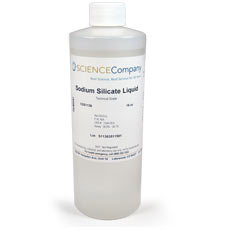An image of a tall, cylindrical plastic bottle with a slightly off-white, light gray color and a screw-on white plastic cap. The bottle features a white label that prominently displays the text "Science Company" in unreadable colors at the top, and "Sodium Silicate Liquid" in black below it. Although the rest of the text on the label is too small to read, it is clear that the simple design aligns with a scientific aesthetic. The bottle appears mostly clear, making it challenging to ascertain the liquid level, though it seems nearly full just above the label. The bottle casts a small shadow at its base, and the overall background is a plain white, making the image focused solely on the bottle itself.